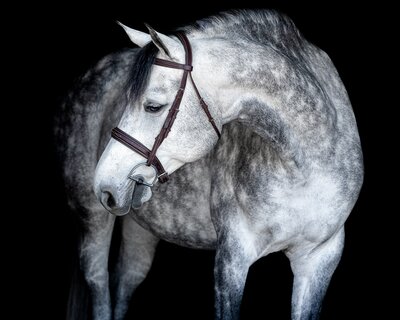This artistic depiction presents an elderly, large horse predominantly in shades of white and gray with subtle charcoal accents, standing upright against a stark black background. The horse's head is turned backwards towards the left, revealing its expressive black eyes and black nostrils. Its coat is primarily white with patches of gray and darker charcoal tones, more prominent around its underbelly, face, and ears. A piece of darker hair peeks between the horse's ears, while the inner parts of the ears and the mouth feature darker charcoal hues. A brown leather rein loosely encircles the horse's neck, highlighting the detailed artistry of the piece. The style of the image, which could be watercolor, pencil, oil-based painting, or digital art, emphasizes the central, gracefully twisted position of the horse, adding to its enigmatic and contemplative demeanor.